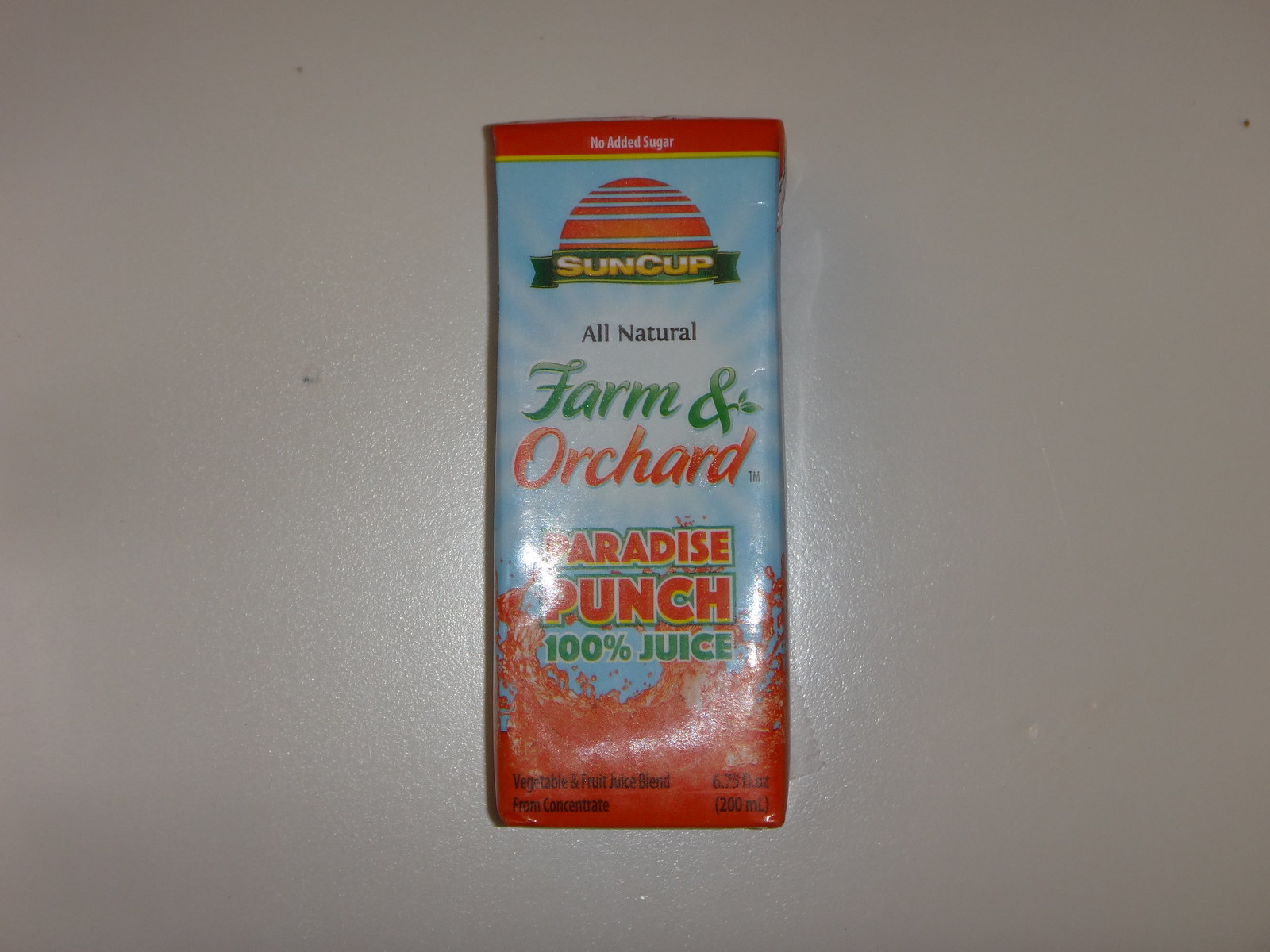The image features a plastic pouch of juice against a white background. The top of the pouch is designed with a half-circle red section, interspersed with several blue marks. The middle of the pouch showcases a prominent red rectangle that indicates there is "No Added Sugar." The bottom of the pouch is green, and within this section, the brand name "Sun Cup" is clearly visible. The pouch touts its content as "All Natural" and specifies that the juice is from "Farm and Orchard." The flavor of the juice is "Paradise Punch," and it is labeled as "100% Juice," with the liquid inside appearing to be a mix of green and red. The bottom-right corner of the pouch states the volume as "6.75 fluid ounces (280 milliliters)." Light reflection off the plastic makes the letter "P" somewhat hard to see on either side, and the bottom-right area of the pouch is brightly illuminated.